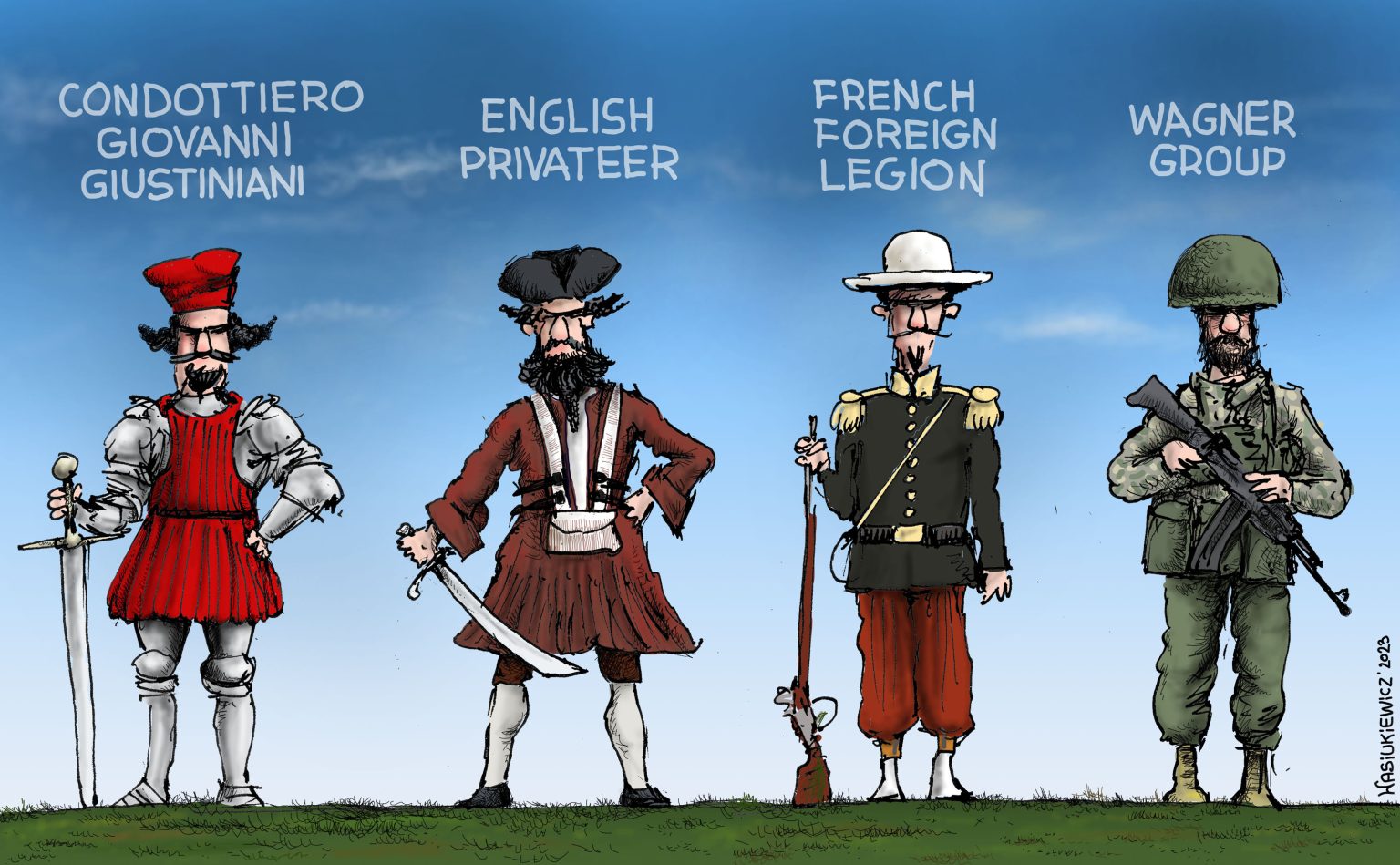This detailed illustration showcases caricature drawings of mercenaries through different periods in history. Starting from the left, it features Condottiero Giovanni Giustiniani, depicted in full body armor with a red turban, goatee, and a sword resting on the ground by his feet. Next is an English privateer, illustrated with a pirate hat, full beard, and dressed in a brown coverlet with a pouch. Following him is a French Foreign Legion soldier in a typical uniform with a rifle resting on the ground, adorned with striped orange pants and epaulettes on his shoulders. Finally, on the right is a modern-day Wagner Group mercenary, equipped in full military fatigues, combat boots, a helmet, and carrying an AK-47. These caricatures effectively capture the evolving image of mercenaries, who serve as private fighters throughout varying historical contexts.